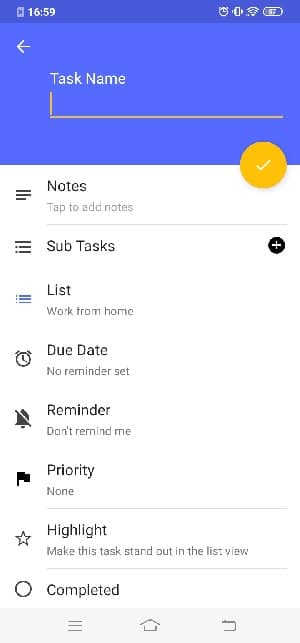This image depicts a digital screen, characterized by poor quality with noticeable blurriness, fuzziness, and pixelation. At the top of the screen, a blue background can be seen. Positioned on the left-hand corner, the time reads "16:59". To the right, there are several icons aligned from left to right: an alarm clock, a vibration symbol, a Wi-Fi signal, and a battery indicator. Directly beneath the blue section, on the left side, is a white arrow pointing to the left along with the text "Task Name" beneath it. A gray horizontal line runs across the screen under this section. Toward the right, a check mark encircled by yellow is visible. The lower portion of the screen features a white background, segmented into several tabs. From top to bottom, the tabs are labeled as follows: "Notes," "Subtasks," "Lists," and "Due Dates."